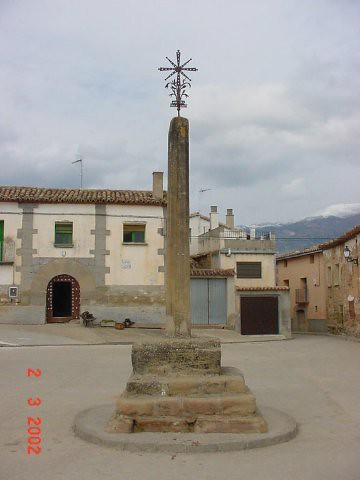This color photograph, taken in portrait orientation, captures a historic South American monument set in a barren courtyard. The image, approximately three to four inches tall and two and a half to three inches wide, prominently features a stone obelisk that is as tall as a person. The obelisk, made of beige or brown stone, stands in the center of the image atop a base composed of three stone steps, creating a stepped or staircase effect, and a raised circular platform of light brown dirt. At the obelisk's peak is an intricate ornamental cross with an overlaid X design. Surrounding the courtyard are older stucco buildings with slanted, red-tiled roofs and arched doorways, characteristic of the region's architectural style. The skyline is filled with cloudy gray skies, and a snow-capped mountain range rises in the background on the left side. In the lower left-hand corner, vertically printed in orange, the date reads "2-3-2002."